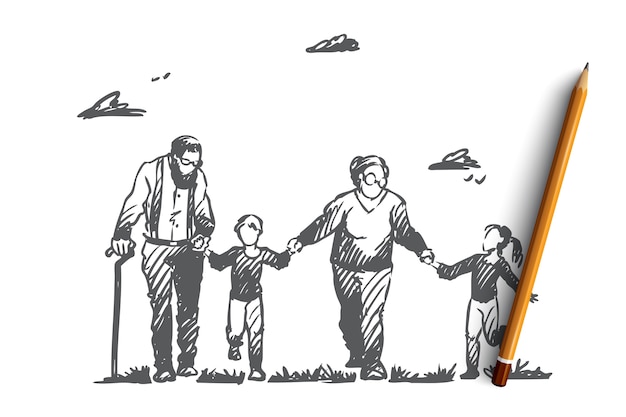This illustration depicts a minimalistic, monochrome sketch of a family of four—comprising a grandfather, a grandmother, and their two young grandchildren—walking together. The entire scene is rendered in what appears to be pencil or pencil-like digital strokes, against a white background, with shades of grey enhancing the details. Puffy clouds and a few birds populate the sky, while a ground layer of simple grass is sketched beneath the figures' feet. The characters, devoid of facial details, are distinguished by their attire and posture. 

The grandfather, positioned on the left, is identifiable by his glasses, beard, and cane. He wears suspenders over a striped shirt and pants and has brown hair. He holds the hand of a little boy who is connected in turn to the grandmother. She is outfitted in a sweatshirt, pants, and round glasses, with her hair pulled back in a bun. The grandmother holds the hand of a little girl on her right, who looks up at her. This girl has her hair in a ponytail and wears a long-sleeved shirt. A striking element of the image is a sharp, yellow pencil placed diagonally across the little girl's outstretched left arm, adding a meta-layer suggesting the act of drawing itself. Despite its minimalistic style, the sketch evokes a warm, familial connection amidst a serene outdoor setting.